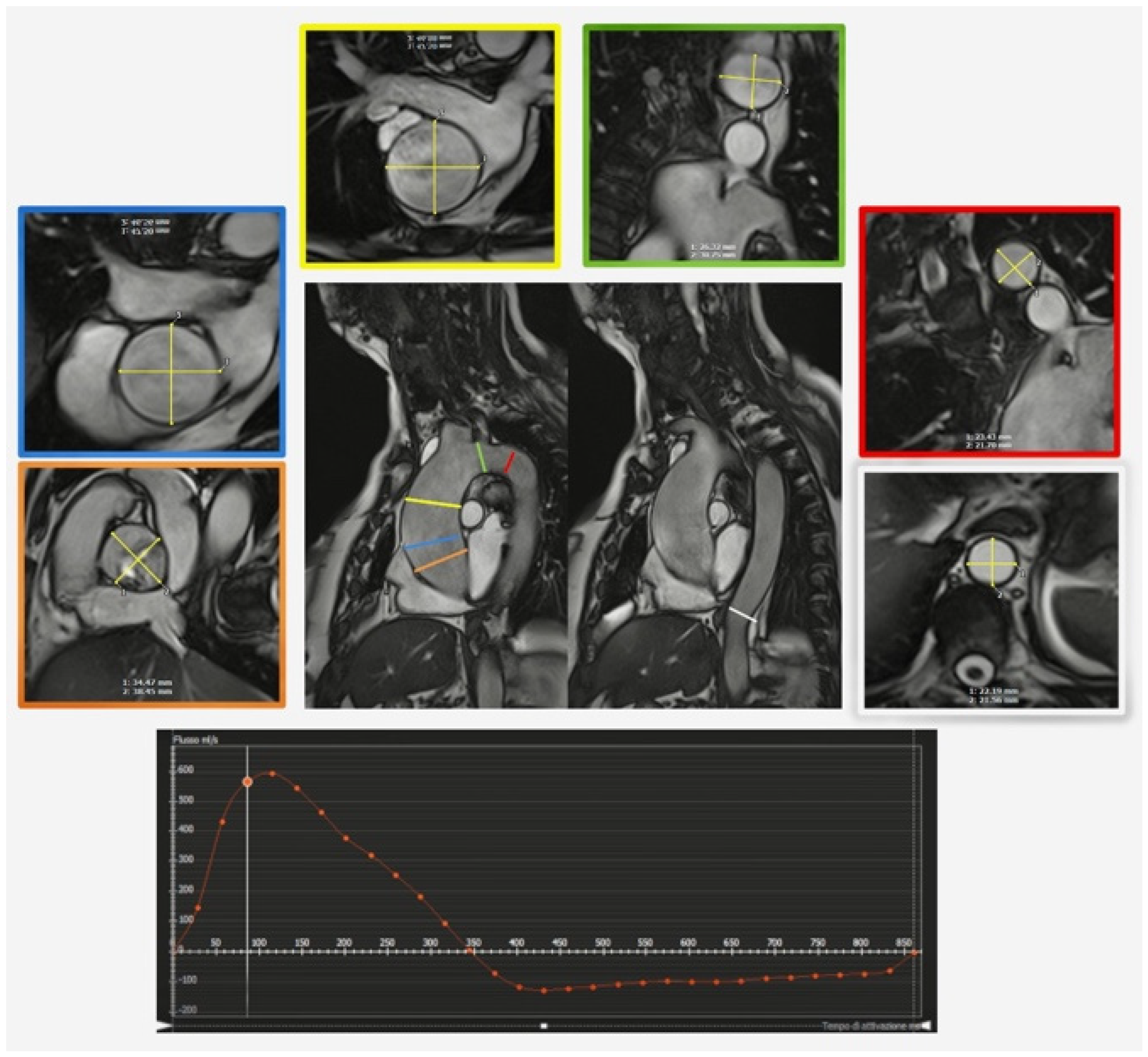The image is a detailed medical imaging report resembling abstract art at first glance. It features six small x-ray photos arranged on the top, both on the right and left sides, with the central area dominated by a large x-ray showing a cross-section of the neck and chest. The borders of these images are vivid and varied, including colors such as blue, orange, yellow, lime green, red, and gray. Each x-ray is annotated with colored markings, such as yellow, green, blue, orange, and red, to highlight specific areas. The central image has four lines pointing towards what appears to be the heart, drawn in red, green, yellow, blue, and orange. Below these x-rays is a black-background graph featuring white numbers and a red plotted line that descends dramatically below the number lines. All the images are displayed on a white background, and there is no additional text aside from the numbers on the graph.